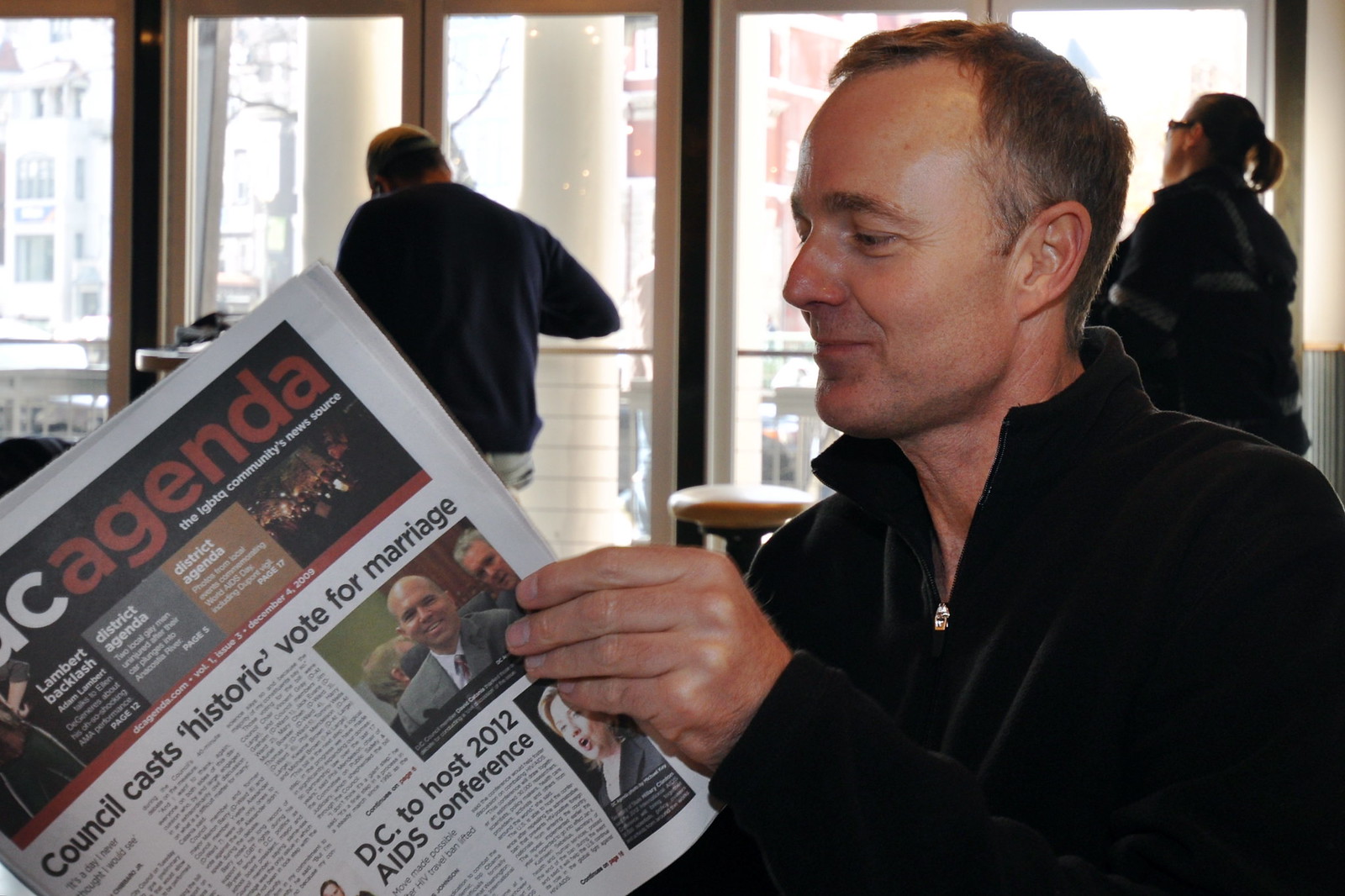In the image, a casually dressed man with short brown hair is reading a newspaper or magazine while seated in what appears to be a cozy coffee shop or restaurant. He seems to be enjoying the content, wearing a long-sleeved black quarter-zip sweatshirt. The newspaper's front page showcases the headline "Council Casts Historic Vote for Marriage", with the word "Agenda" prominently displayed in red, though the full name is cut off. Below the headline, another article reads "DC to host 2012 AIDS Conference." The setting includes tall floor-to-ceiling windows, possibly doors, revealing buildings and cars outside, including a noticeable white building and a red building. The interior shows a stool in the center, and behind the man, a woman in a black jacket stands near the windows gazing outside while another gentleman in a blue jacket and beige pants sits at a table. The scene captures an inviting and lively atmosphere, with the focus on the man engrossed in his reading.